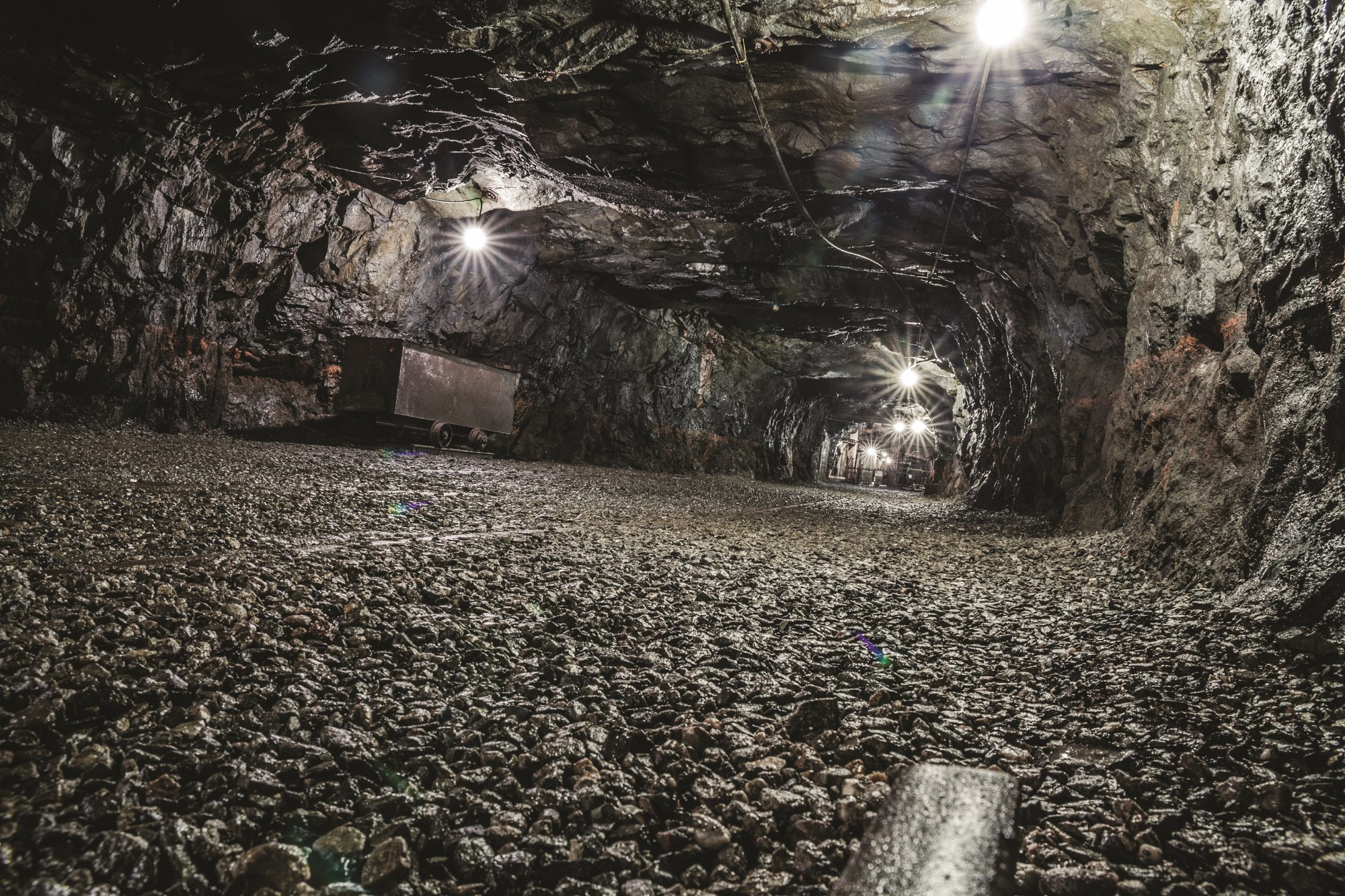This photograph captures a dimly lit underground cave, displaying a tunnel with rugged, mottled dark gray stone textures enveloping the floor, walls, and curved ceiling. The image is taken from a low, ground-level perspective, adding depth to the scene. A faint, rusty mine cart rests on tracks to the left side of the frame, near the foreground, with its two small wheels clearly visible. The mine cart is positioned against the left stone wall, which continues to form an arch over the tunnel.

Bright white lights, some with noticeable lens flares, are suspended from the ceiling at regular intervals, illuminating the otherwise dark and shadowy passage. These lights are connected by visible piping that runs along the top of the cave. Toward the distant end of the tunnel, additional lights and what appear to be cages are faintly visible, subtly outlining the extent of the passage. The overall monochromatic palette of grays and blacks in the photograph accentuates the cave's rough texture and the age-worn features of the mining equipment within.